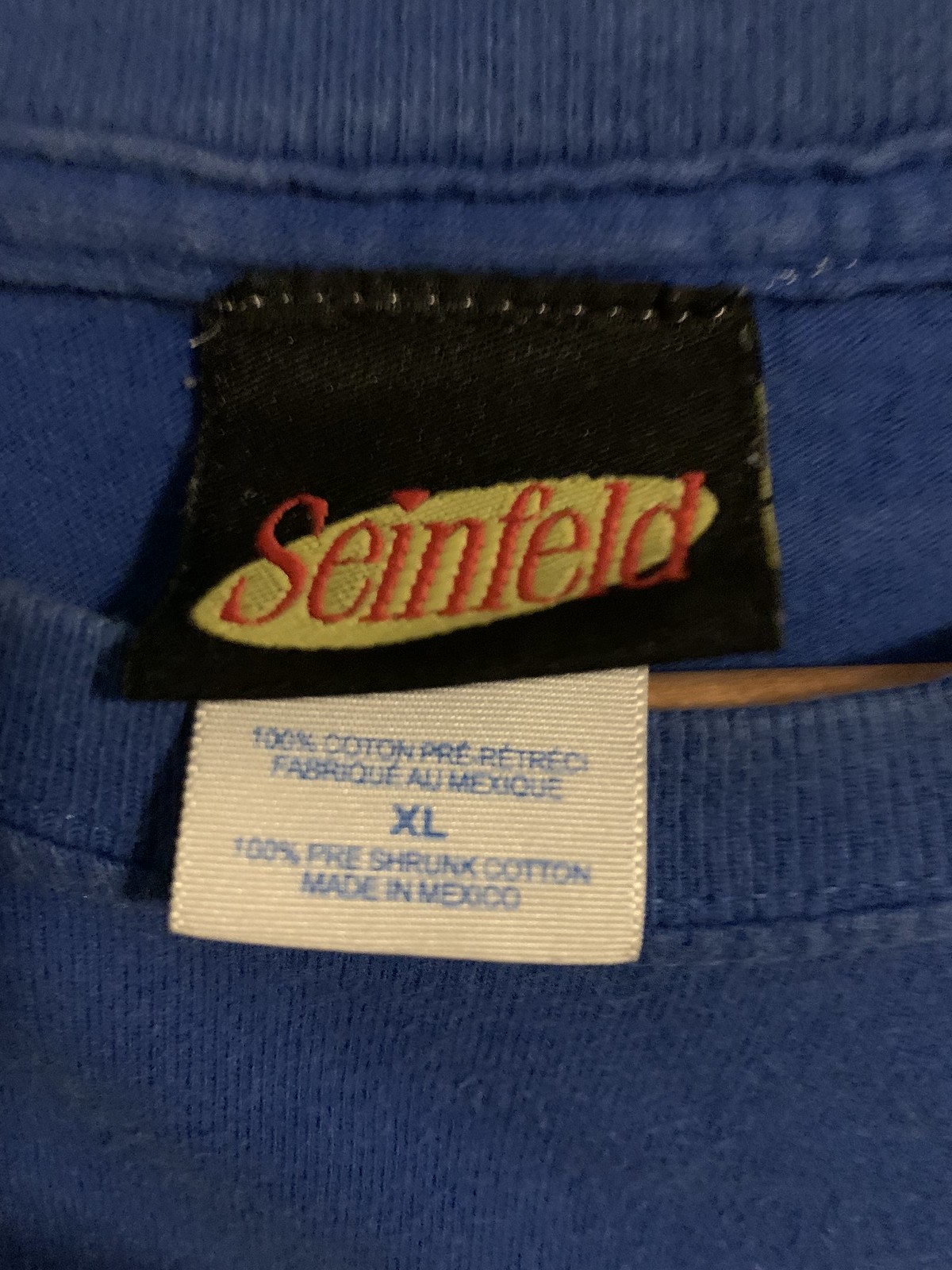Close-up photo of a medium blue denim sweatshirt featuring two tags. The first tag is black with an elongated oval in a tannish-gold color. Inside the oval, "Seinfeld" is embroidered in dark pink thread. Below this tag, there is a white, ribbed ribbon tag bearing text in both English and French. It reads: "100% cotton," followed by "C-O-T-O-N," "Pre-r-e-t-r-e-c," "F-a-b-r-i-q-u-e-a-u," and "M-e-x-i-q-u-e," indicating that the sweatshirt is made in Mexico. The tag also mentions the size: "Extra Large," with the additional note: "100% pre-shrunk cotton made in Mexico."